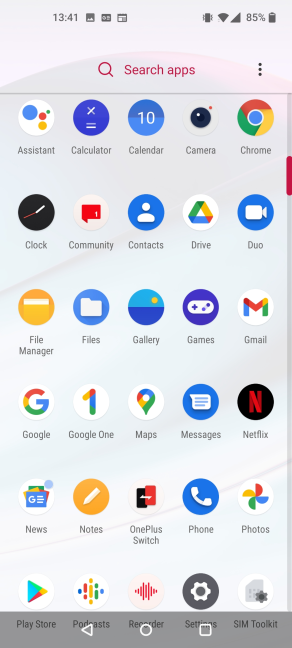This image, in portrait orientation, presents a standard cell phone screen displaying all installed apps against a light gray backdrop with a subtle swoosh pattern. At the top left corner, the time is displayed as 13:41 alongside three small icons. To the right, traditional cell phone indicators show that the phone is on vibrate mode, connected to Wi-Fi with full signal bars, and the battery is at 85% charge. Below these indicators, centered in magenta text, is a search bar labeled "Search apps" accompanied by a magnifying glass icon to its left. To the right of the search bar, three vertical dots in dark text are visible.

The main section of the screen features a grid comprising five columns and six rows of app icons. The apps are listed as follows:

**First row (left to right):** Assistant, Calculator, Calendar, Camera, Chrome.
**Second row:** Clock, Community, Contacts, Drive, Duo.
**Third row:** File Manager, Files, Gallery, Games, Gmail.
**Fourth row:** Google, Google One, Maps, Messages, Netflix.
**Fifth row:** News, Notes, OnePlus Switch, Phone, Photos.
**Sixth row:** Play Store, Podcasts, Recorder, Settings, SM Toolkit.

At the very bottom of the screen, there's a gray navigation bar featuring three central white icons: a left arrow, a circle, and an outlined square.